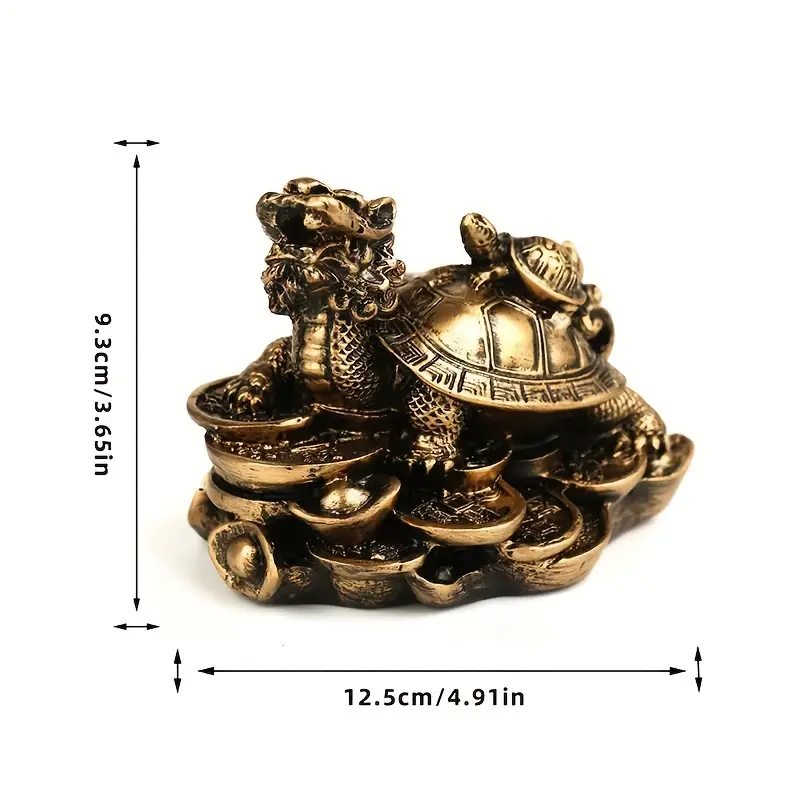The image showcases a detailed, gold-colored metal object set against a white background, with precise measurements indicated on the sides. On the left side, there's a vertical arrow pointing up and down, with "9.3 cm / 3.65 inches" printed nearby. At the bottom, a horizontal, two-way arrow points left and right, displaying "12.5 cm / 4.91 inches" underneath. At the center, the object depicts a fascinating structure: a large turtle-like body with a shell, crowned by a smaller, traditional turtle. Interestingly, the larger turtle's head resembles that of an Asian dragon, with an open mouth and intricate detailing, suggesting a blend of mythical and animalistic features. This composite creature stands atop a series of layered, large circular trays or coins, giving an impression of a fountain or a stack of oversized coins. The entire piece appears to be a single, meticulously soldered metal trinket, possibly of historical or decorative significance.